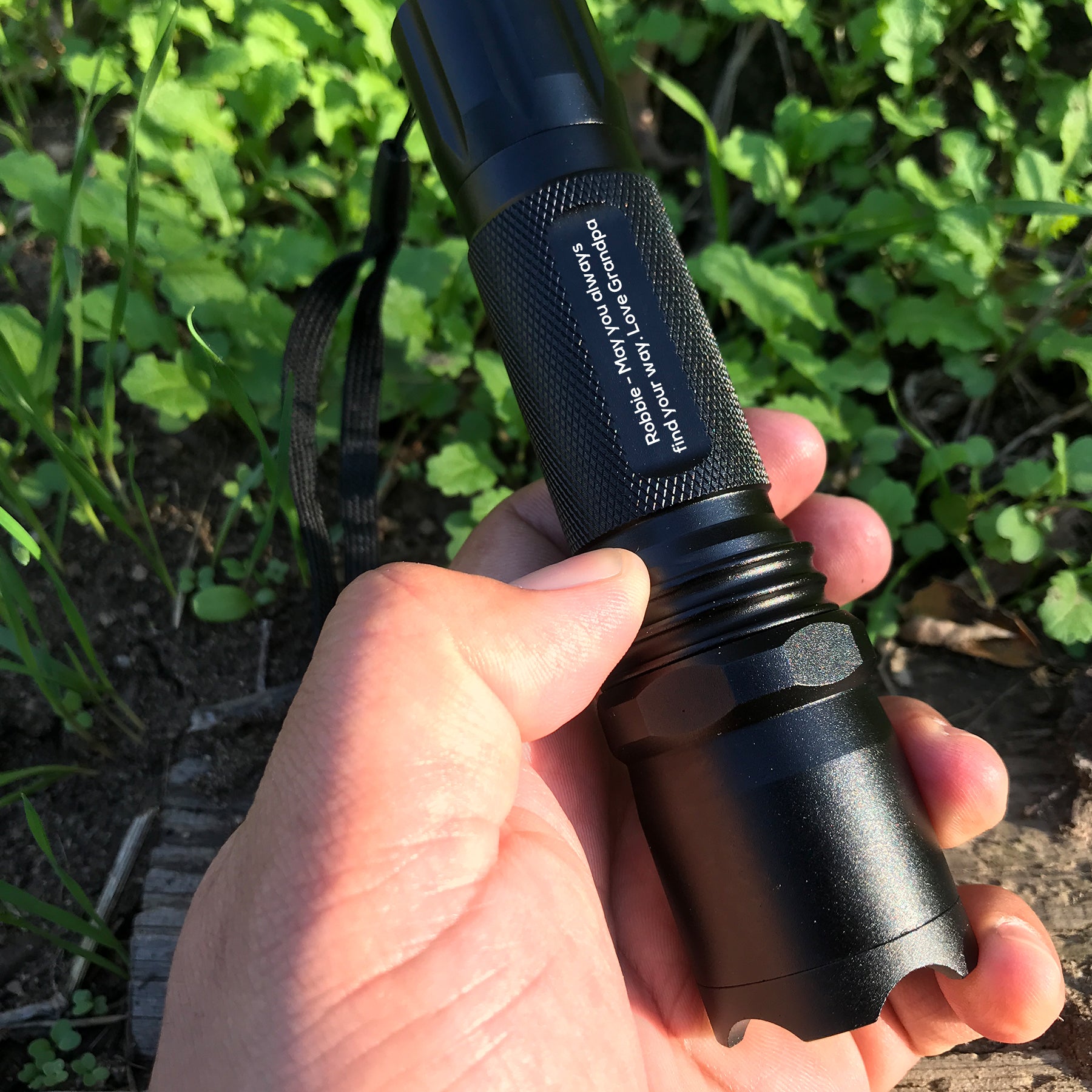In this detailed photograph taken outdoors during the day, a clean, white left hand is prominently displayed, holding a modern black metal tactical-style flashlight. The hand, visible from the bottom, tightly grips the flashlight with wrapped fingers and thumb, emphasizing a secure hold. The flashlight, which exudes a strong, contemporary technical appearance, features an engraving in delicate white lettering that reads, "Robbie, may you always find your way. Love, Grandpa." This heartfelt message marks the flashlight as a personalized item, possibly seen in a catalog or advertisement. The engraved text is small but clearly visible on the flashlight’s sleek black surface. A fabric lanyard is attached to the flashlight, imparting both a tactical and utilitarian vibe. The backdrop consists of a lush hedge or shrub with large, green leaves in varying shades, accompanied by a hint of gray, somewhat resembling a log or stone, situated at the bottom left corner of the hedge, adding depth and context to the natural outdoor setting.